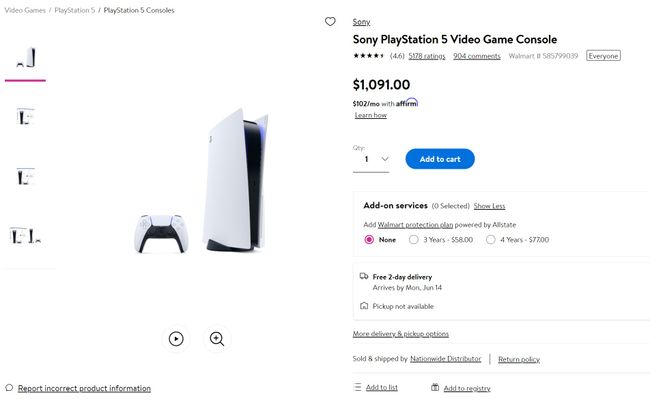This image is a detailed screenshot of a product page on Walmart's website for a Sony PlayStation 5 video game console. On the left side of the screenshot, there is a main image displaying a stock photo of a white PlayStation 5 console accompanied by a matching white controller. To the left of this main image, there are four smaller thumbnail images arranged vertically. The top thumbnail is identical to the main image and features a purple bar beneath it indicating its selection. The remaining thumbnails appear to show different angles of what is presumably the console's packaging, though the details are too small to discern clearly.

On the right side of the screen, there is a shopping information area. This section includes:
- The product title
- A star rating for the product
- The price, which is listed as $1,091, or alternatively, $102 per month through Affirm financing
- A quantity selector, currently set to one unit
- A prominent blue "Add to Cart" button with white text
- An add-on services section that offers protection plans from Walmart. This section includes three radio button options: "None" (which is currently selected with a purple circle), a three-year plan for $58, and a four-year plan for $77, both of which are grayed out and unselected.
- A delivery information section that promises free two-day delivery with an expected arrival by Monday, June 14th. This section also mentions that pickup is not available, includes an icon of a truck, and has additional small text detailing delivery options and list/registry additions.

Overall, this comprehensive product page layout provides all the necessary details a customer might need when considering the purchase of a PlayStation 5 console from Walmart.